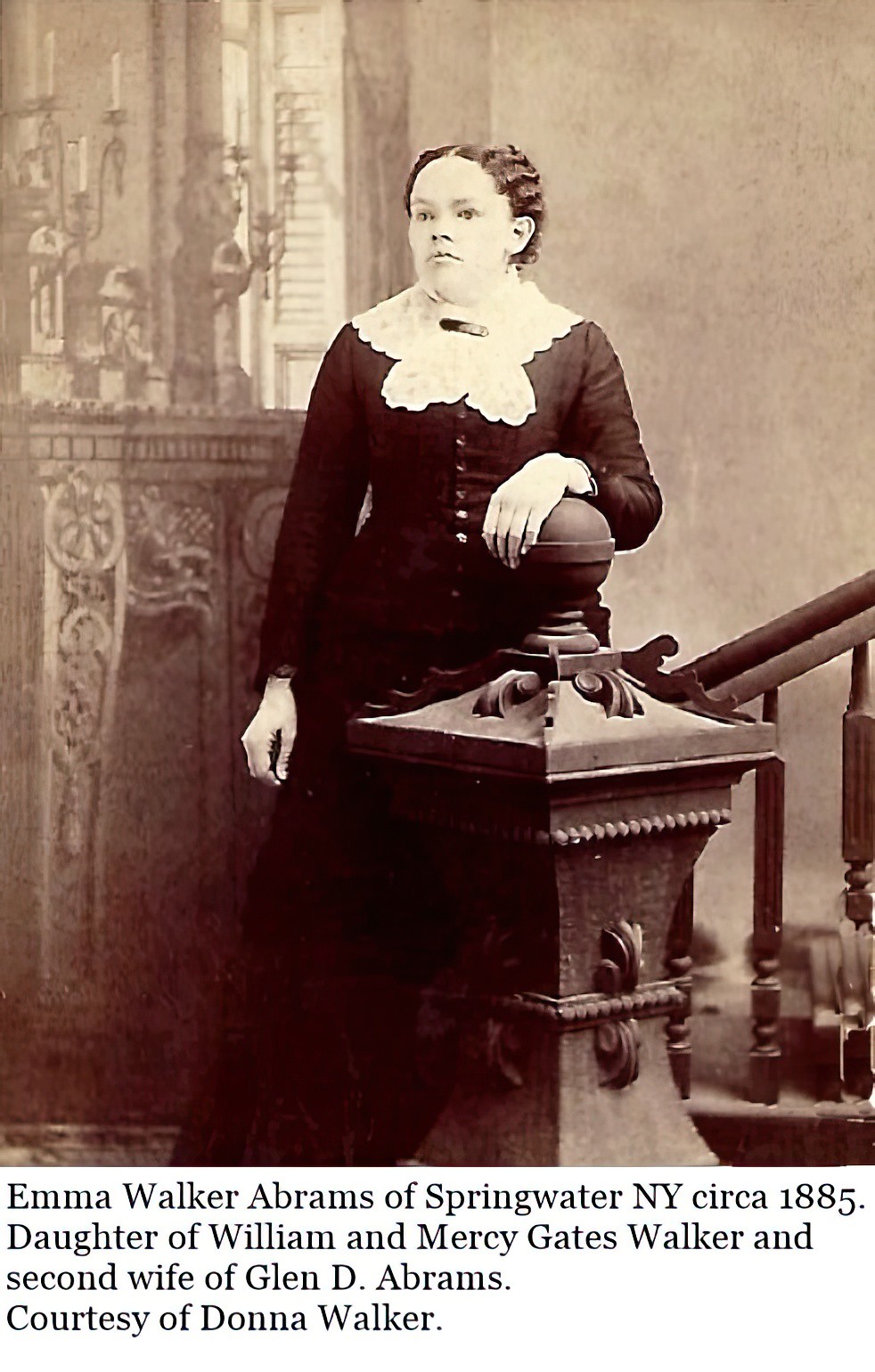This vintage black-and-white photograph, taken circa 1885, features Emma Walker Abrams of Springwater, New York, the daughter of William and Mercy Gates Walker, and the second wife of Glendy Abrams, courtesy of Donna Walker. Emma stands at the base of a staircase, resting her left hand on an ornate pedestal post. Her attire is traditional and modest, clad in a long black dress with a buttoned-up front and a white lace collar wrapped around her neck. She has a somber expression on her puffy face, with her hair styled in a pulled-back fashion. The setting includes a wall behind her with candlesticks placed on an ornate ledge to the left and a tapestry visible in the background. The photograph, complete with its descriptive caption in black text on a white background, exemplifies the intricate detail and formal attire characteristic of the late 19th century.